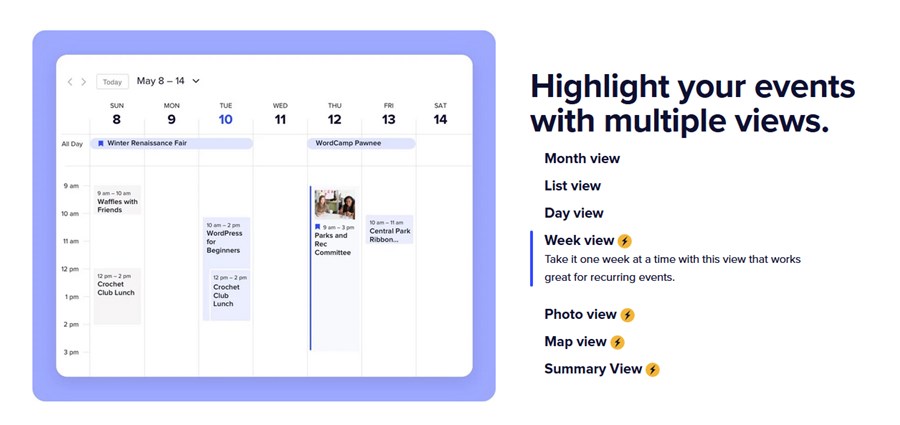Screenshot of a web page featuring a calendar planner interface. On the left side, outlined in a blue box, is a calendar highlighting several events for the week. Some of the notable entries in the calendar include:

- Sunday, the 8th: "Winter Renaissance Fair" (all day), "Waffles with Friends" (9 AM - 10 AM)
- Tuesday, the 10th: "Crochet Club Lunch" (12 PM - 2 PM)
- Thursday, the 12th: "WordCamp Panay" (9 AM - 2 PM) and "Parks and Rec Committee" (10 AM - 12 PM) taking place in the "Central Park Room"

The right side of the page contains descriptive text, introducing features to highlight events using various view options. These include:

- Monthly list view
- Day view
- Week view, noted with a lightning bolt in a yellow circle, indicating its efficiency for recurring events
- Photo view
- Map view, each marked similarly with a lightning bolt in a yellow circle, signifying special functionality
- Summary view also highlighted with a lightning bolt

The overall interface has a white background with black text, providing a clean and user-friendly experience for organizing and managing events effectively.